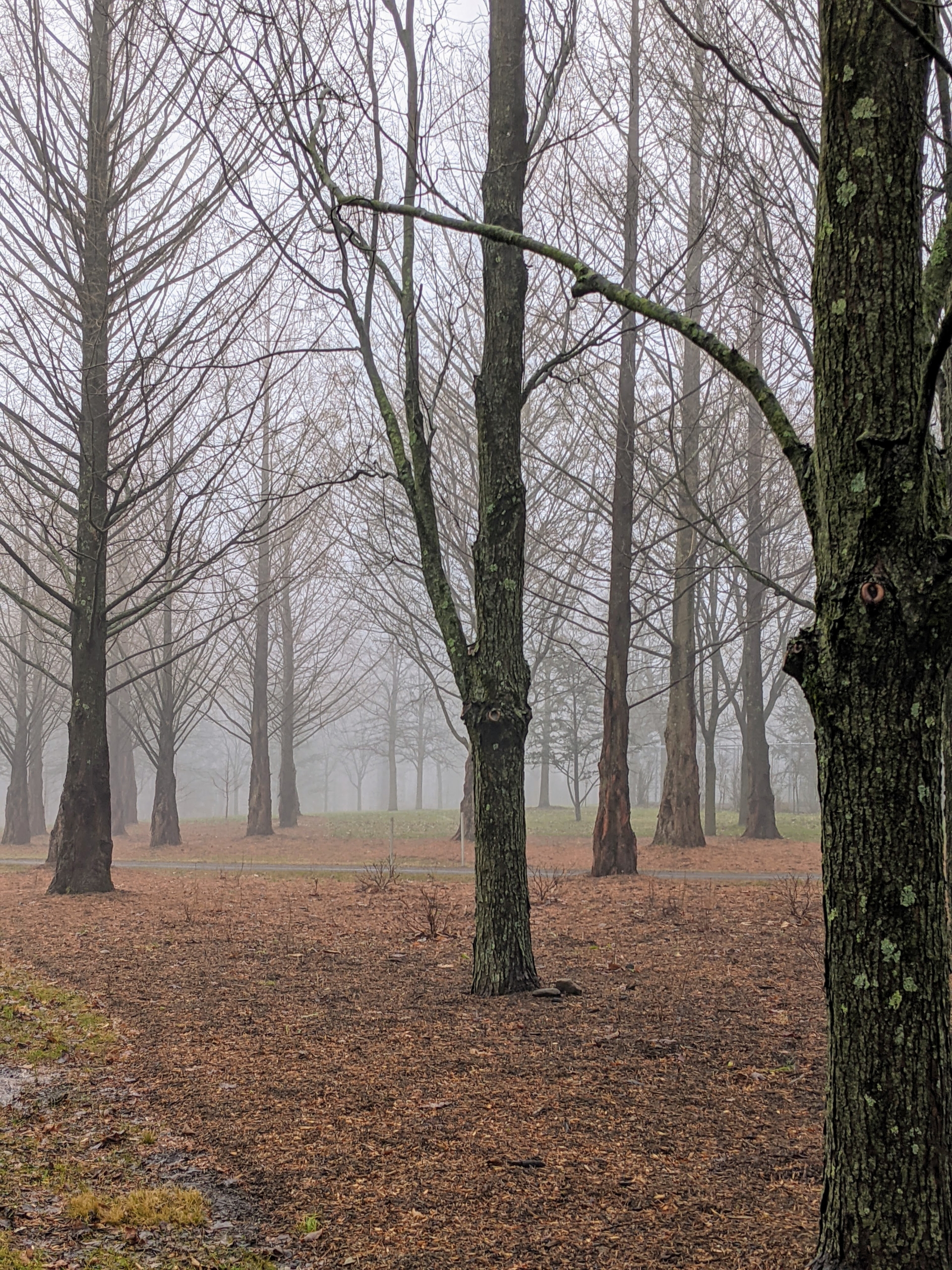The photograph depicts a dense forest area, likely taken during autumn or early winter. The scene is populated with numerous tall trees, all devoid of leaves, revealing their bare, brown trunks and long, spindly branches. The forest floor is carpeted with fallen brown leaves and patches of moss, adding to the earthy tones of the scene. In the center, a roadway or path bisects the forest, leading the eye into the distance. The day is foggy, with a visible mist that blurs the further trees, giving the background an ethereal, hazy quality. The grass transitions from a tan color in the foreground to patches of green farther back, suggesting a change in elevation or moisture levels. The overall atmosphere is one of quiet solitude, with the fog and leafless trees creating a serene, almost otherworldly, woodland scene.